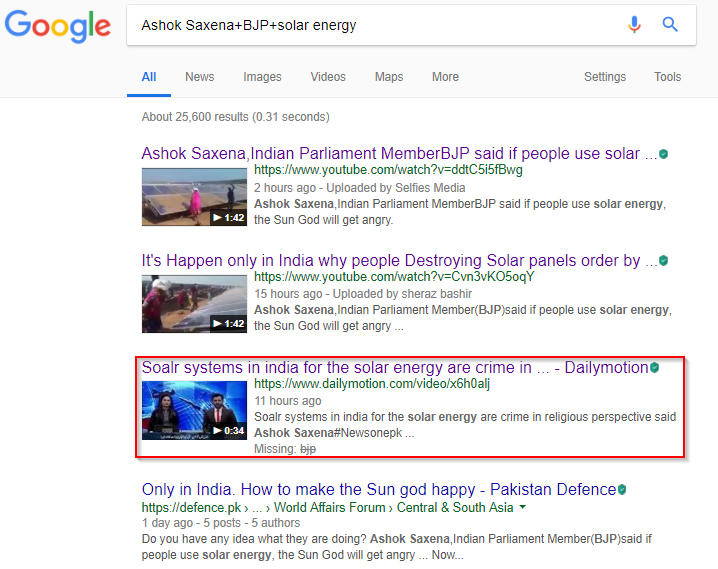This detailed caption describes a Google search results page focused on a specific topic concerning an Indian parliamentary member and solar energy:

The image shows a Google search results page categorized under "Websites." The search query entered is "Ashok Saxena BJP Solar Energy." At the top, you can see the familiar Google search interface with options like "All," "News," "Images," "Videos," "Maps," "More," "Settings," and "Tools." Alongside the search bar, there are icons for voice-to-text input (microphone) and the search button (magnifying glass).

The primary search result highlights Ashok Saxena, an Indian Parliament Member from the BJP, making a controversial statement. The headline of the featured result states that Ashok Saxena said if people use solar energy, the "sun god will get angry." This result links to a YouTube video, which was uploaded just two hours ago by Selfies Media.

Below this, the next search result is a news article or blog post titled, "It's Happened Only in India: Why People Destroying Solar Panels?" This content reiterates the parliament member's statement that the use of solar energy could anger the sun god. Additionally, it discusses the notion that using solar systems in India may be considered a crime from a religious perspective. Another link below this content suggests a related topic, "Only in India: How to Make the Sun God Happy," sourced from Pakistan Defense.